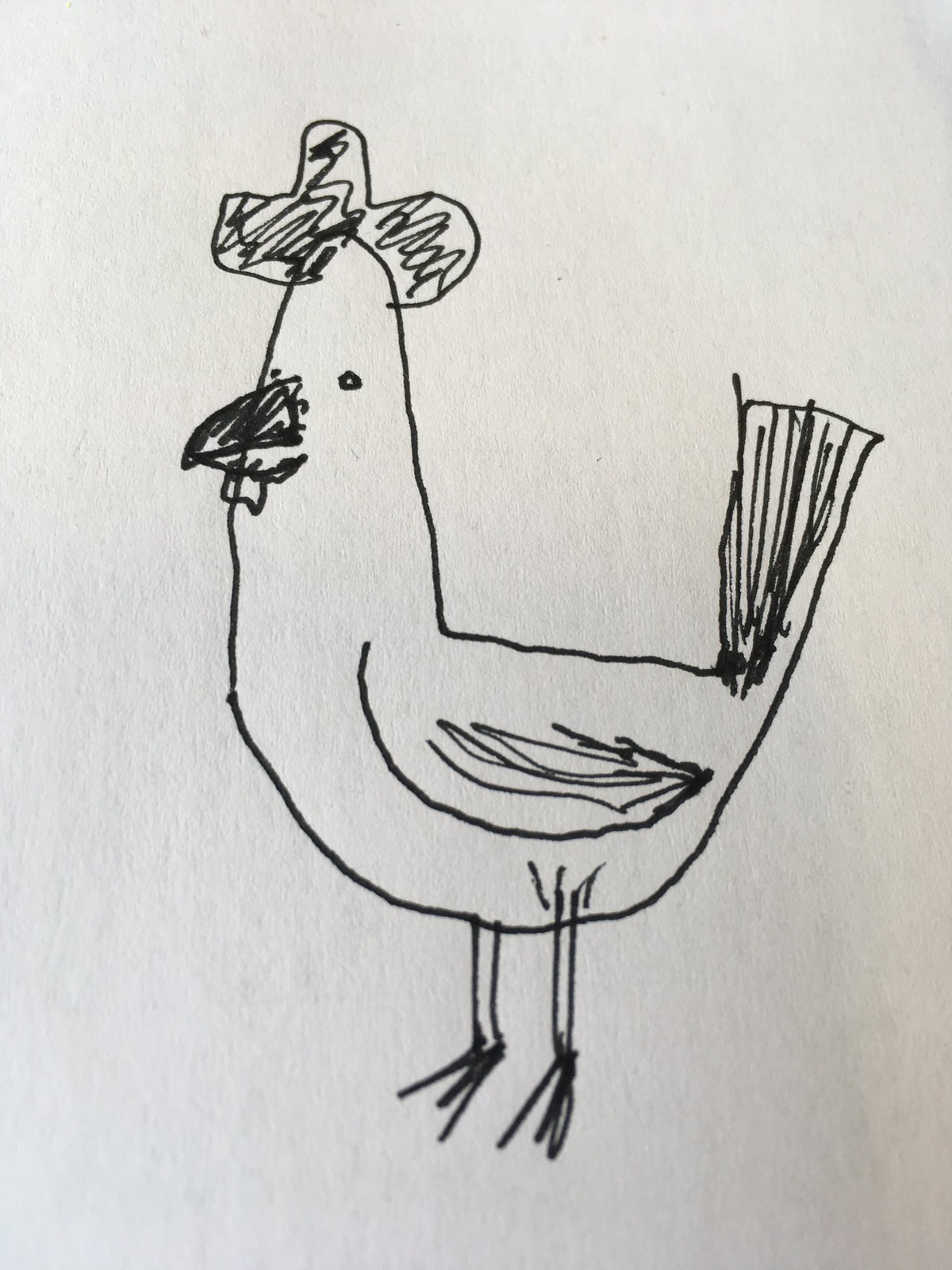The image features a photograph of an off-white, almost light gray sheet of paper with a crude, simplistic drawing created by an inexperienced artist using a black marker. The drawing depicts a bird, likely meant to represent a rooster or a chicken, positioned facing left. The bird has a basic rounded body and stands on two spindly legs with stick-like feet.

Its head, located on the left side of the drawing, is adorned with a hat that might be interpreted as a cowboy hat or sombrero, crudely scribbled and only partially filled in. The bird’s red comb, represented by three bumpy shapes filled with squiggles, sits atop its head. The beak is composed of two curved triangles converging, with the top half shaded in through black scribbles, and a small circular dot represents its eye.

The bird’s wing is simply outlined with a few lines, and its tail sticks straight up, filled in with similar black lines. The lower part of the photograph is slightly blurry, capturing the texture of the paper and a reflection of a light source in the lower left, making this part of the paper appear brighter. Overall, the drawing exudes a whimsical and rudimentary charm, characteristic of an artist's early attempts at sketching.